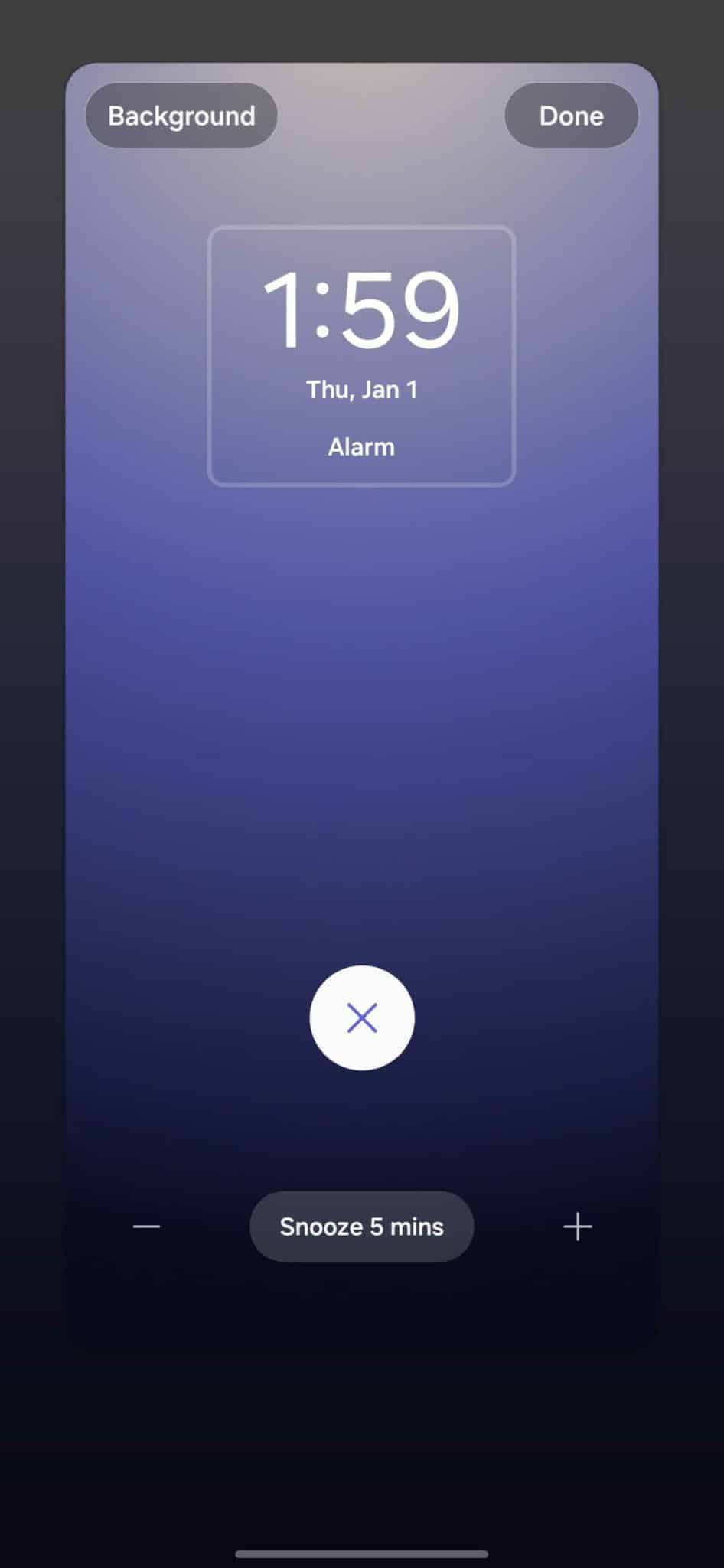A cell phone screenshot is displayed, illustrating an alarm interface. In the upper left corner, there's a gray button labeled "Background," and in the upper right corner, another gray button labeled "Done." Between these buttons, the time "1:59" is shown in white, below which it states "Thursday, January 1st" alongside an indication that this is an alarm, though it is unclear if the time is AM or PM.

Centered below the date and time text, there is a white circle featuring an "X" symbol, likely intended to close the screen. Beneath this, at the bottom of the screen, there are three buttons: a minus sign on the left, a "Snooze 5 minutes" button in the middle, and a plus sign on the right. All these elements are also white.

The background of the interface starts with a white color at the top near the "Done" and "Background" buttons, gradually transitioning to blue and then to black towards the bottom. The phone itself is encased in a border that begins as gray at the top, blending into darker gray, then blue, and finally dark blue to black at the bottom.